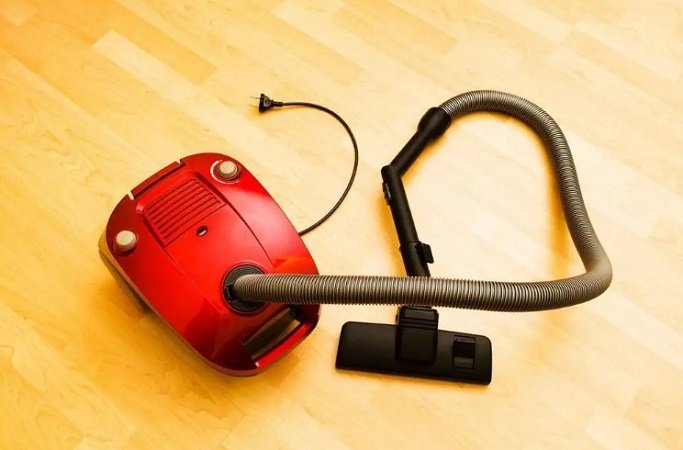The image captures a top-down view of a vacuum cleaner set on a bright, light-colored hardwood floor. The floor's tones range from yellowish to beige, giving it a slightly golden appearance. The vacuum cleaner itself has a striking red base with two prominent beige buttons on either side, each about an inch in diameter. A black wire plug is visibly protruding from the red base. Extending from the front of the vacuum cleaner is a dark brown, coiled hose, twisted somewhat, indicating that the vacuum isn't standing completely upright. The hose curves up, then down, and ends with a black vacuum head that features a venting mechanism. This detailed setting suggests a household environment where the vacuum is ready for use to clean the floor.